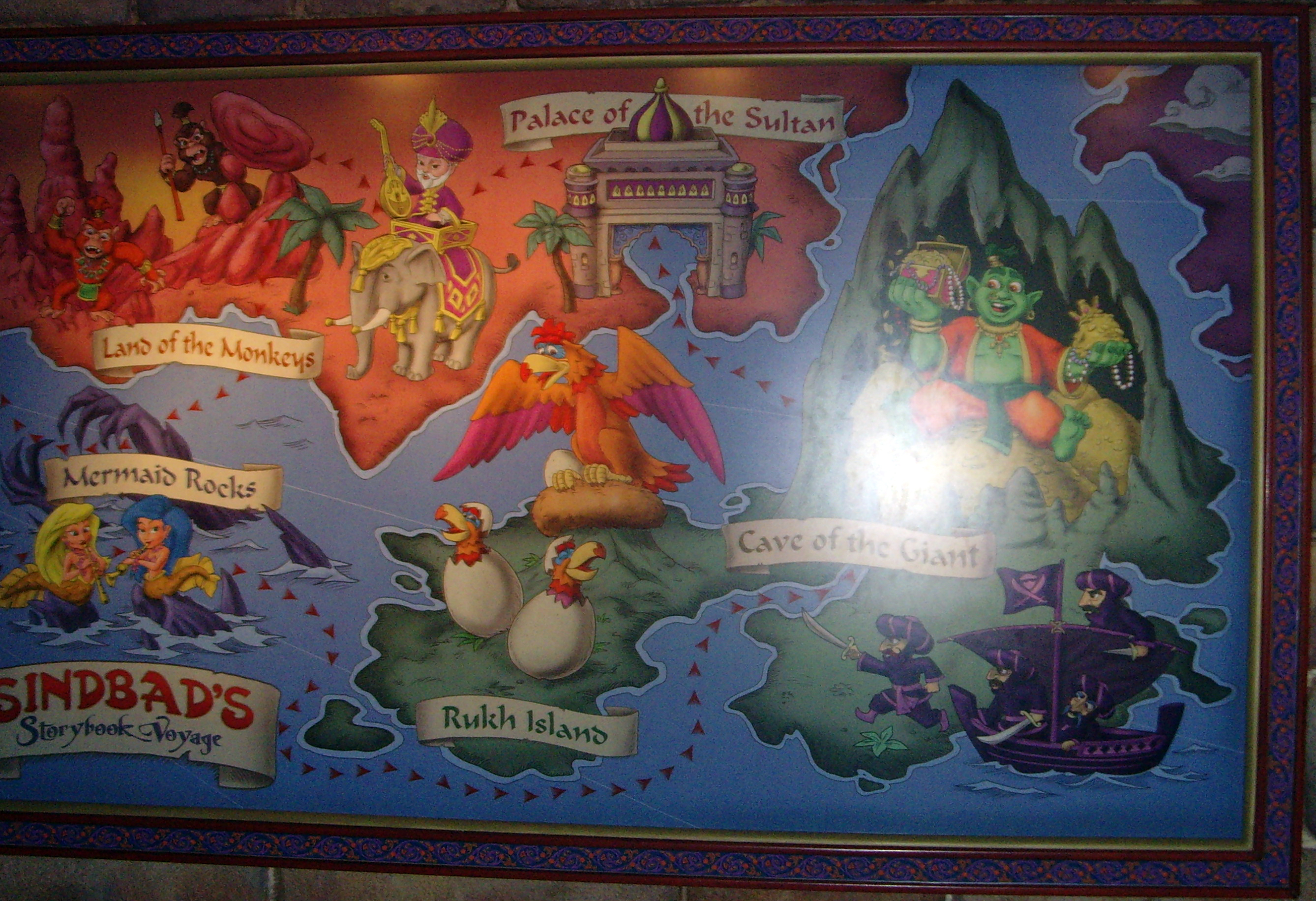This vibrant map poster, titled "Sinbad's Storybook Voyage," is a fascinating blend of fantastical elements and detailed illustrations. The backdrop, a vast expanse of blue, represents the surrounding waters, accentuating different labeled landmasses teeming with characters.

Near the bottom, a lush green area labeled "Rock Island" features a large bird with two hatching eggs and a pair of pirates advancing with swords. Notably, trolls are also present, adding to the mystical atmosphere. To the left, within the waters, marked as "Mermaid Rocks," two mermaids sit serenely on rocky outcrops, while mysterious fists or claws protrude from the depths.

On the upper section, a landmass is identified by the inscriptions "Palace of the Sultan" and "Land of the Monkeys." This area shows a man riding an elephant alongside a monkey wielding a spear, set against a backdrop of towering mountains and elaborate figurines. Additionally, another section known as "Cave of the Giant" is depicted with a genie surrounded by a treasure trove of jewels, alongside more playful details like birds and exotic animals, creating a rich tapestry of Sinbad's legendary voyages.